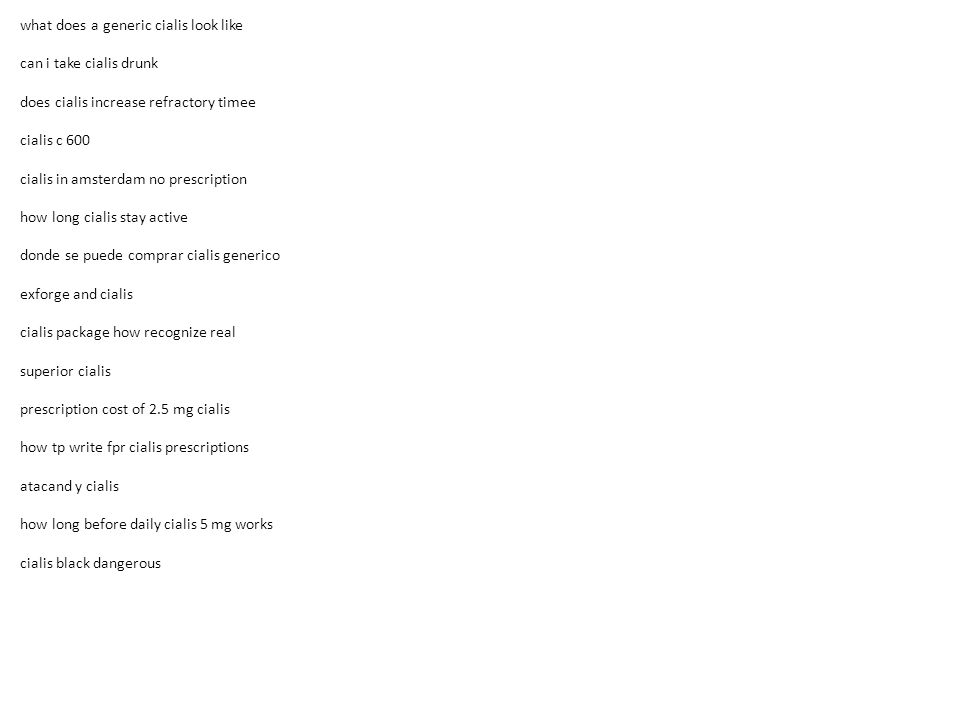The image depicts a section of a website dedicated to providing information about a type of medication, likely Cialis. The webpage features a clean, white background with a comprehensive list of various topics related to Cialis, presented in small black font on the left side of the page. 

The listed topics cover a wide range of questions and statements, including:
- "What does generic Cialis look like?"
- "Can I take Cialis drunk?"
- "Does Cialis increase refractory time?"
- "Cialis C600"
- "Cialis in Amsterdam no prescription"
- "How long does Cialis stay active?"
- A section in Spanish
- "Xforge and Cialis"
- "Cialis package: how to recognize real"
- "Superior Cialis"
- "Prescription cost of 2.5 milligram Cialis"
- "How to write a prescription for Cialis"
- "Atacan and Cialis"
- "How long before daily Cialis MG works?"
- "5 MG and Cialis black dangerous"

The webpage appears to offer detailed information and possibly FAQs to help users understand various aspects of Cialis, from its physical appearance to its usage, effectiveness, and related prescriptions.